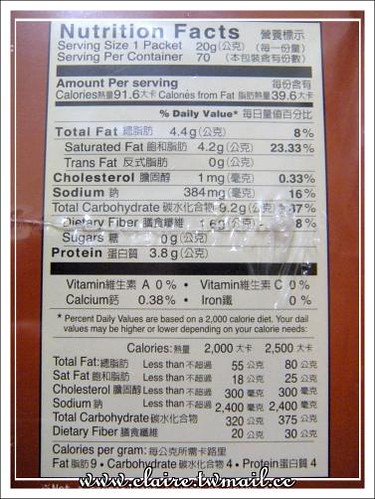This image showcases the Nutrition Facts label on the back of a food product package. The background of the label is white with black text, bordered by a burgundy-colored edge. The label, detailing nutrients in both English and Chinese, specifies that the serving size is one packet (20 grams) and the container holds 70 servings. The nutritional breakdown per serving includes: 91.6 calories, with 39.6 calories from fat. Detailed component values are listed—Total Fat: 4.4 grams (8%), Saturated Fat: 4.2 grams (23.33%), Cholesterol: 1 mcg (0.33%), Sodium: 384 mcg (16%), Total Carbohydrate: 9.6 grams (17%), Dietary Fiber: 16 grams (8%), Sugars: 0.9 grams, Protein: 3.8 grams. The label also notes Vitamin A (3%), Vitamin C (3%), Calcium (0.38%), and Iron (0%). Percent daily values are based on a 2,000-calorie diet, with additional information provided on daily values for a 2,500-calorie diet. At the bottom of the label, the website URL www.claire.twmail.cc is displayed in white text.